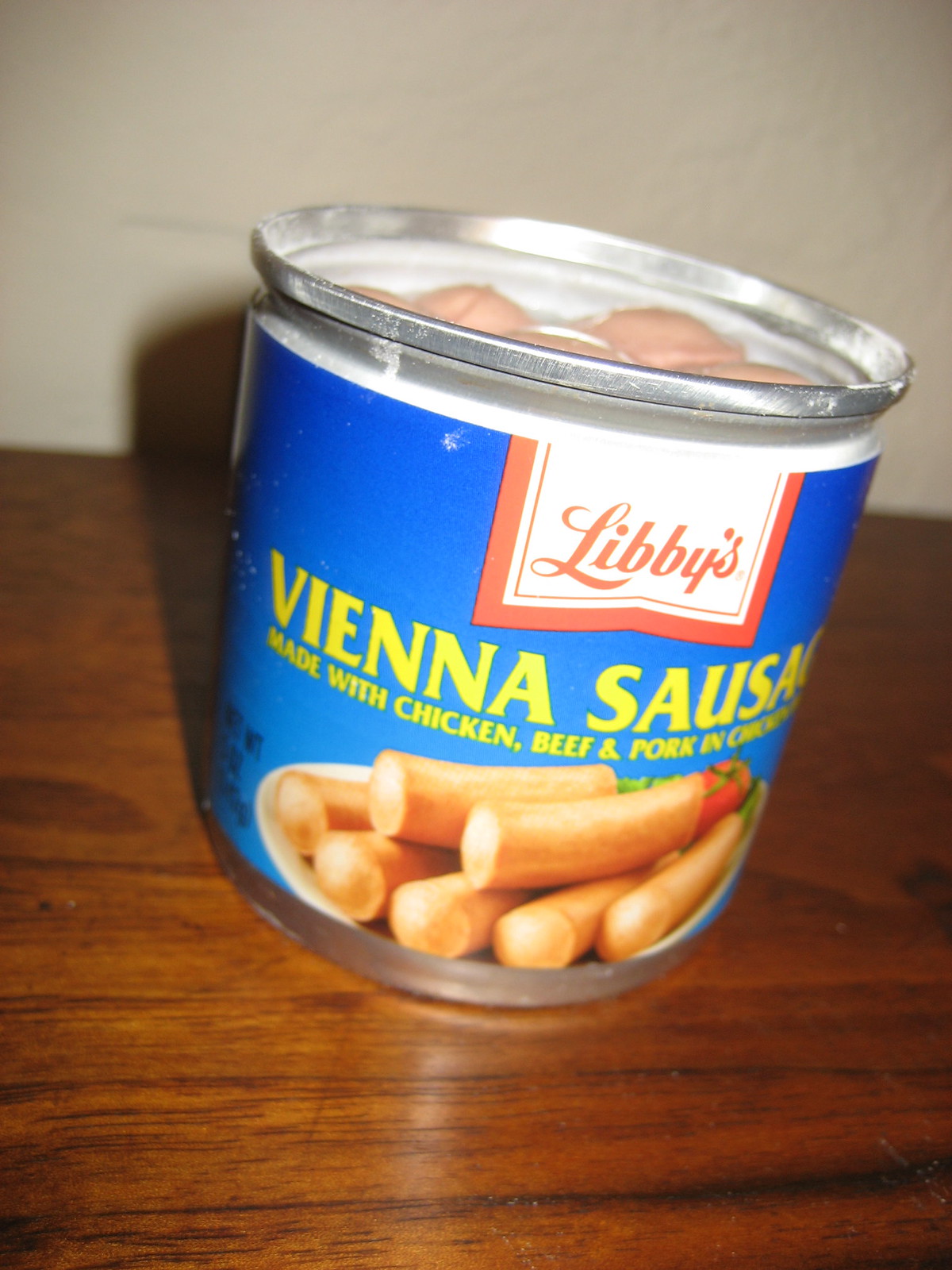A close-up photograph features a small can of Vienna sausage, with the lid already removed to expose the light pink sausages inside. The can is set on a dark wooden table, and the surrounding walls are a white-beige color. The photo was evidently taken at night, as the poor lighting reveals, illuminated mainly by a camera flash.

The can itself has a tin bottom and a blue ombre wrapper that transitions from dark to light blue. At the top of the wrapper is a red and white square with the brand name "Libby's" written in red cursive within the white portion. Below that, in yellow lettering, it reads "Vienna Sausage," followed by text indicating the contents are "made with chicken, beef, and pork," though the last word is partially obscured.

An image on the wrapper depicts a white plate with seven Vienna sausages, arranged with five on the bottom and two on top. A whole tomato and what appear to be peppers are included on the plate, likely to enhance visual appeal. The side of the can, where details such as the net weight are printed, is partly out of view. The flash creates a clear shadow of the can on the table, further emphasizing the scene's dim lighting.